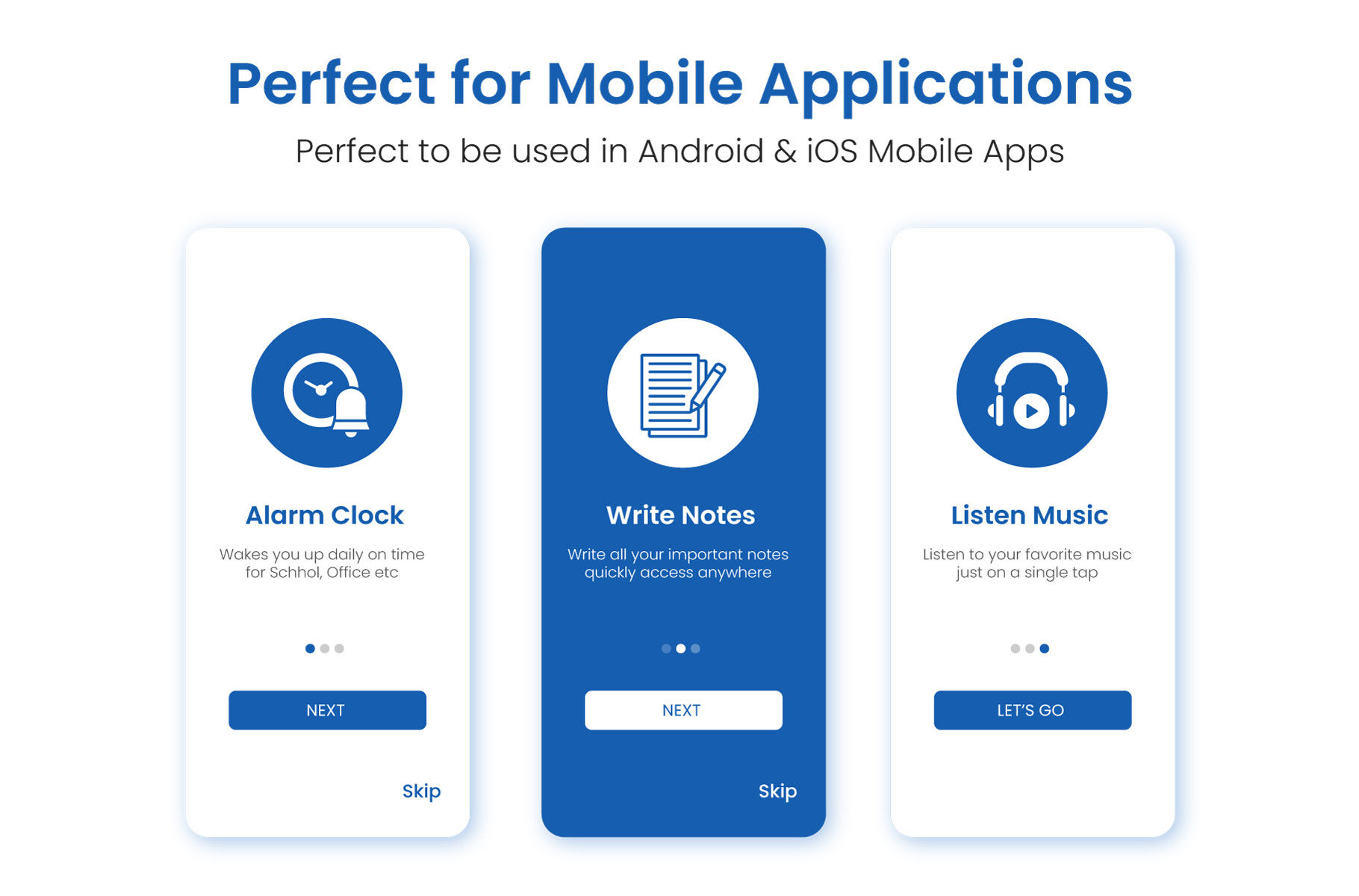The series of images depicts a mobile application designed for both Android and iOS devices. 

1. **First Screen**: The centerpiece is a blue circle containing clock and bell icons, signifying an online alarm clock. This feature ensures users wake up on time for their activities, like school. Below this, there is a blue rectangle labeled "Next", and a "Skip" option at the bottom. The informative visual indicates the app's alarm functionality.

2. **Second Screen**: A blue circle in the center showcases icons like a phone, notepad, pencil, and paper, representing a note-taking feature. Users can jot down important notes easily with this function. This screen also bears "Next" in a white rectangle with blue text and a "Skip" option in the bottom right corner.

3. **Third Screen**: A white rectangle features a blue circle containing headphone and play button icons. This screen highlights the app's music functionality, allowing users to listen to their favorite tracks with a single tap. Below, there’s a "Let's Go" button set against a white background with shadows, hinting at the app's readiness for use.

Overall, this mobile application is presented as a versatile tool for waking up on time, taking notes, and listening to music, making it perfect for both Android and iOS platforms. The consistent shadowing in the background of the images adds depth, enhancing the visual appeal for users across various smartphones.